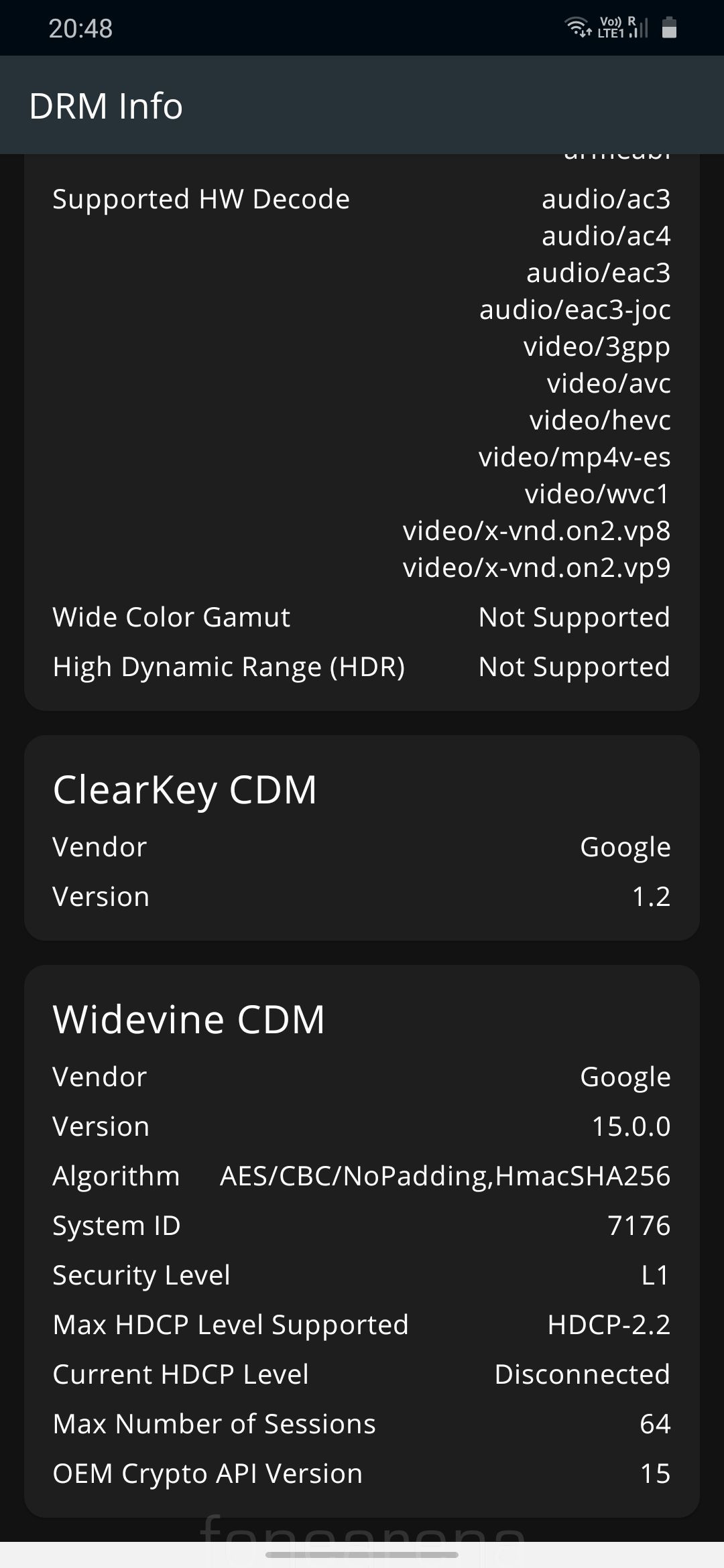This screenshot of a mobile phone display reveals a detailed diagnostic screen filled with white text against a black background, organized into two distinct columns. In the top left corner, the first item listed is "DRM Info." Directly beneath it is the heading "Supported HWD Code," followed by the term "Wide Colour Gamut" with its corresponding status in the right column marked as "Not Supported." Additionally, under the section "Supported HWD Code," the right column lists technical terms such as "Audio/AC3" and "Audio/AC4."

Further down, the term "High Dynamic Range (HDR)" is featured, with the right column again indicating "Not Supported." The next prominent heading is "Clear Key CDM," under which "Vendor" and "Version" are specified. To the right, the vendor is listed as "Google" and the version as "1.2."

Finally, the third section titled "Widevine CDM" completes the diagnostic display, with various features and their attributes outlined in white text. This comprehensive screenshot offers a detailed breakdown of the device's media capability and compatibility specifications.